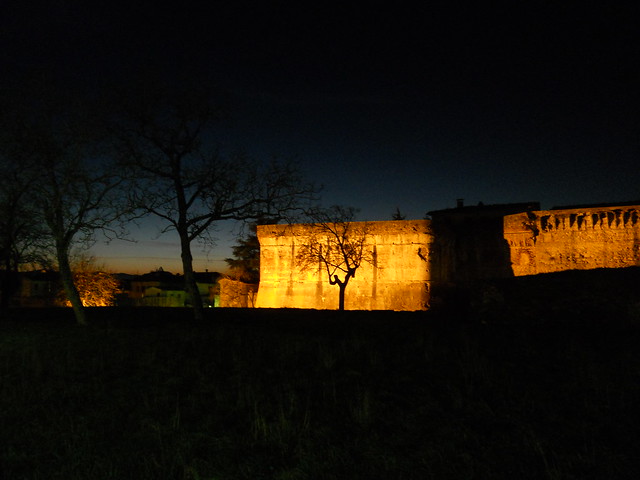This nighttime photograph captures a dramatic scene dominated by a partially illuminated, ancient stone coliseum-like structure. The sky transitions from deep black to shades of blue and a faint orange glow off in the distance, possibly remnants of a sunset or sunrise. The coliseum is highlighted with spotlights, casting an orange and reddish hue on the structure, emphasizing the absence of windows and a smooth, barricaded facade. In the foreground, sparse, jagged trees devoid of leaves frame the scene with stark silhouettes, while one distant tree retains a few brown leaves. The bare trees' shadows stretch across the lit stone, adding depth and intrigue. Behind the coliseum, white houses and additional stone buildings are faintly visible, adding context to the serene yet mysterious nighttime setting. The ground appears dark, obscuring the color of the grass but contributing to the overall ambiance illuminated by artificial light.